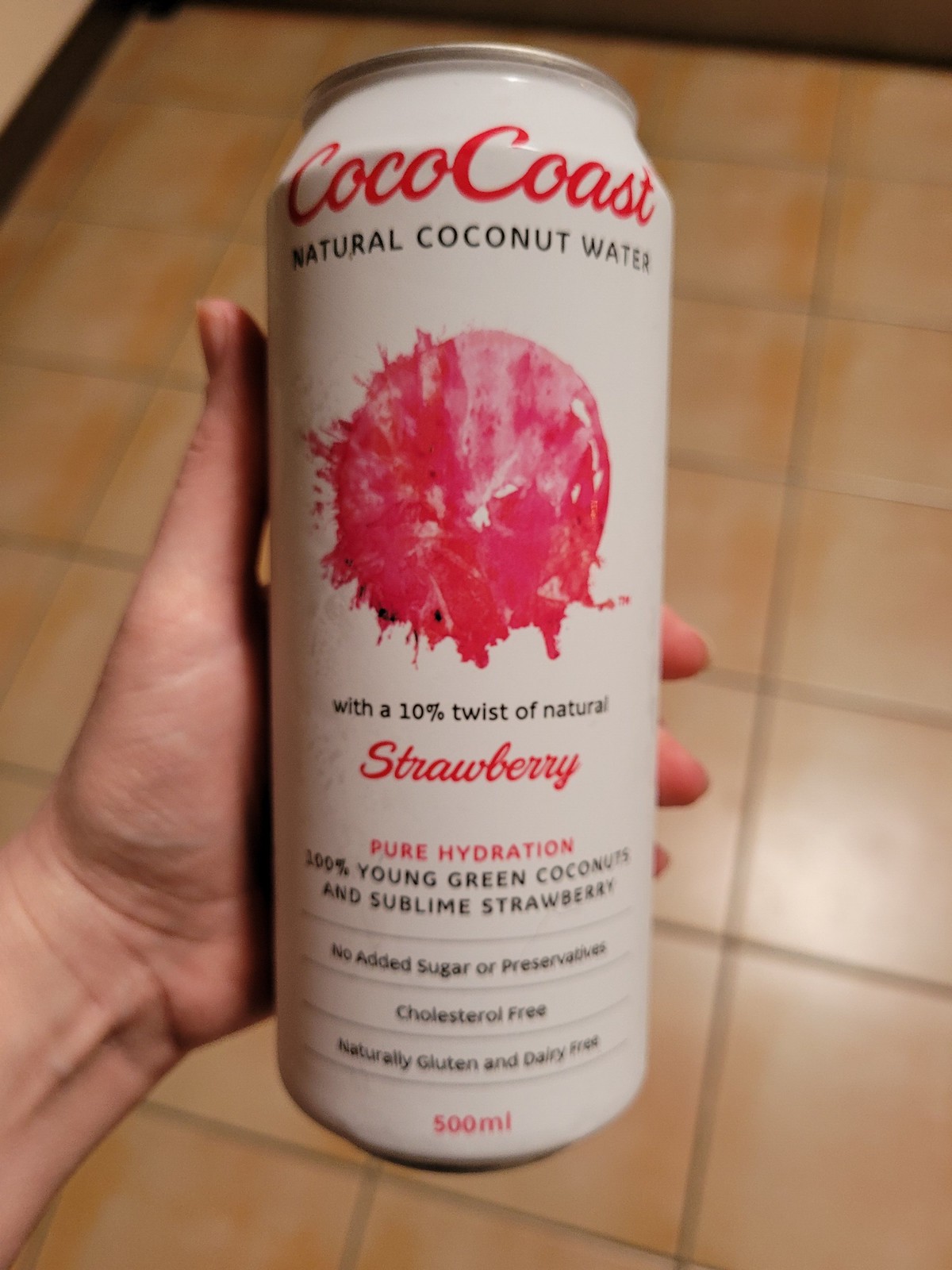This is a detailed photograph of an aluminum can of Cocoa Coast natural coconut water held in someone’s left hand. The can is tall and white, or eggshell-colored, with "Cocoa Coast" written prominently in red script at the top. Below this, in black print, it says "Natural Coconut Water." There is a round, splotchy red design in the center of the can, beneath which it states "with a 10% twist of natural" in black print, followed by the word "strawberry" in red script. Further down, it reads "pure hydration, 100% young green coconuts and sublime strawberry," emphasizing its natural ingredients. Additional information includes "No added sugar or preservatives, cholesterol-free, naturally gluten and dairy-free," and the can's capacity of 500 ml. The hand holding the can is visibly displaying the thumb, the bottom part of the palm, and part of the wrist. Below the hand, a tiled floor is visible, consisting of squares in varying shades of light brown with darker brown tile edges and dark grey grout, adding context to the setting.